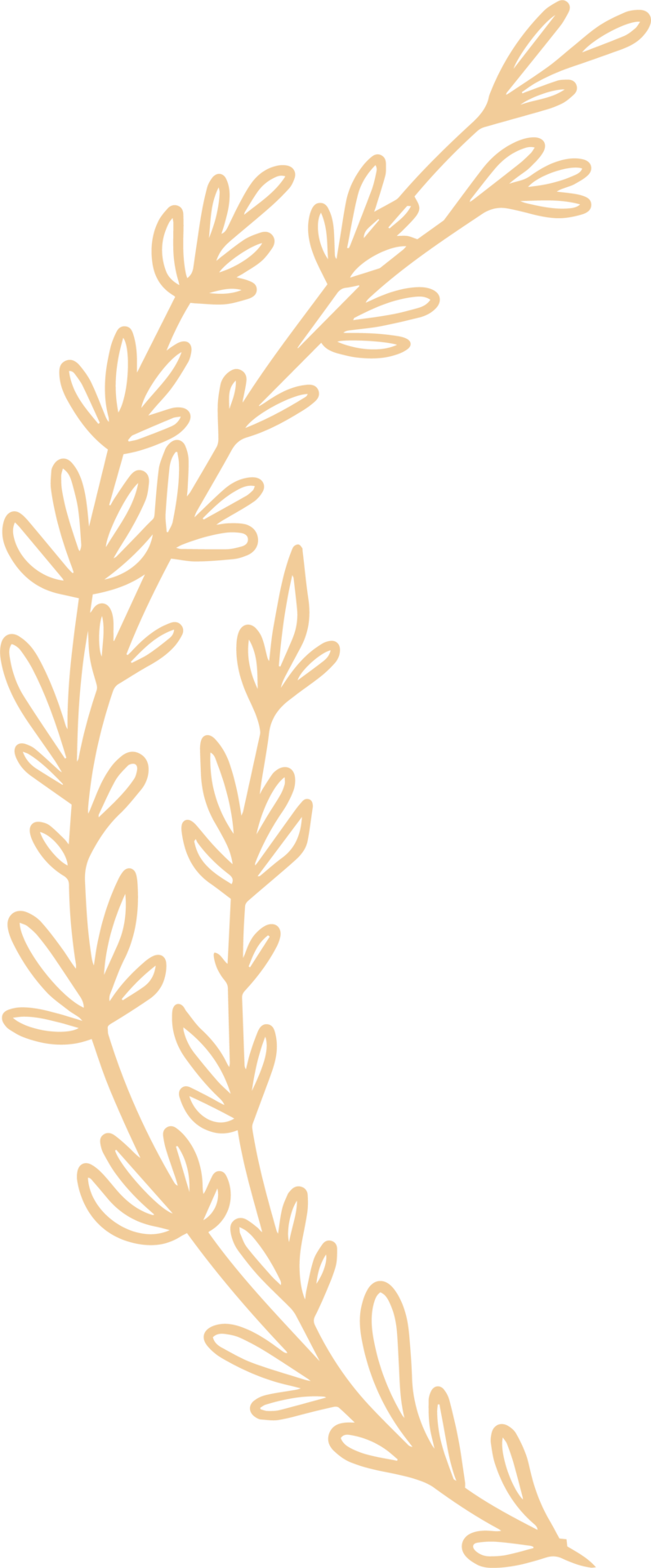The illustration showcases a thyme plant sprig positioned at the center of the image against a plain white background. The plant bends gracefully from the bottom right to the upper right corner, occupying a height of 5 to 6 inches and a width of about 2 inches. The central stem is light brown or tan and arches delicately, splitting into multiple branches along its length. Near the bottom right corner, the stem curves upward, and about an eighth of the way up, it splits into two branches. The right branch extends three-fourths of the way up and features leaves shaped as thin ovals, with the top leaf being the sharpest. The left branch continues upward, splitting again about two-thirds of the way up, with one segment reaching four-fifths of the image height, adorned with five circular points. Each subsequent branch and sub-branch is sparsely dotted with white leaves outlined in brown, contributing to the plant's delicate and detailed appearance. The simplicity of the drawing, with its focus on the elegant curvature and minimalistic depiction of leaves, emphasizes the botanical study quality of the image.